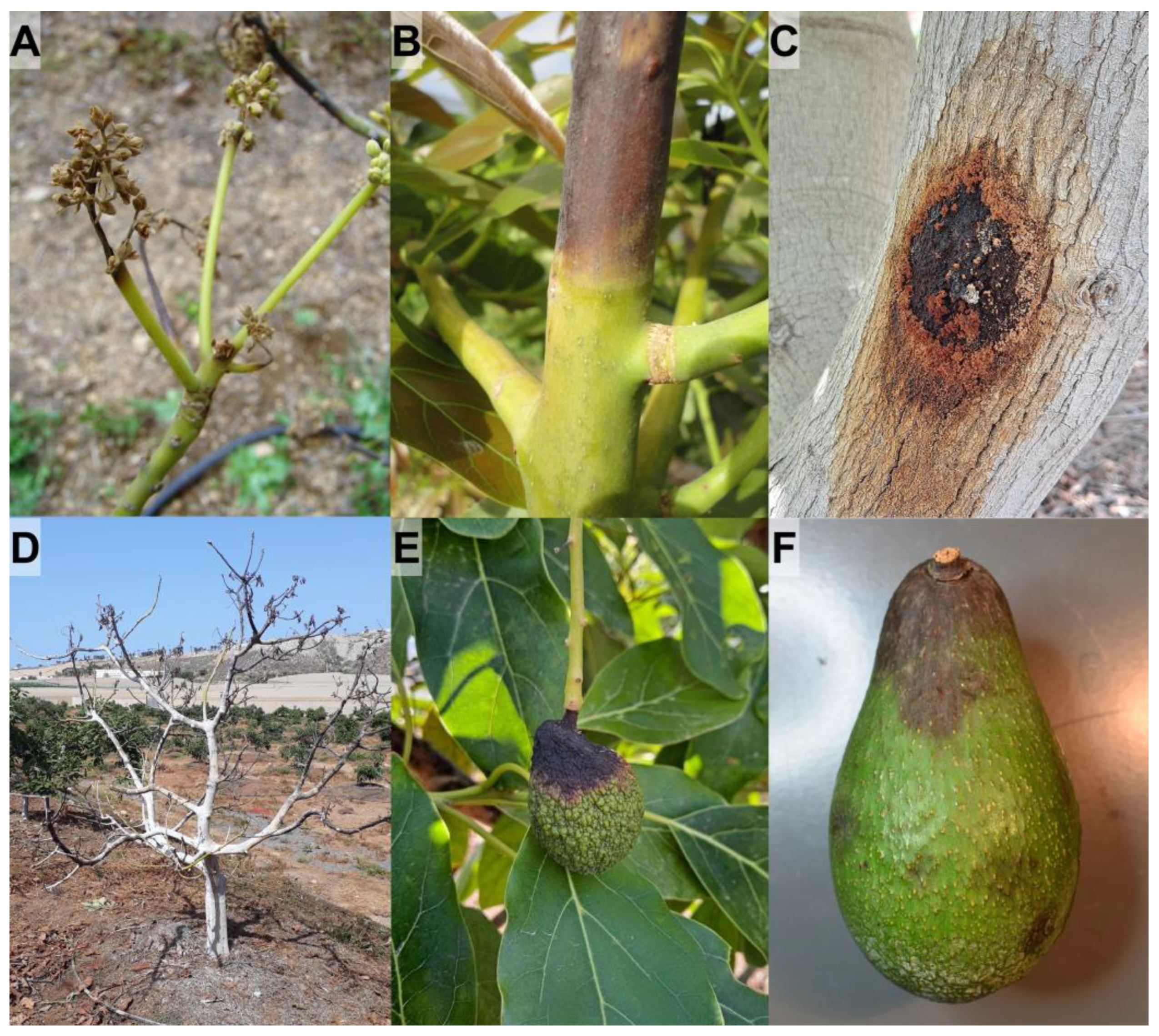This series of six photographs, labeled A through F, illustrates various diseases affecting avocado trees at different stages. Image A shows a wilted avocado flower on the tree set against a background of brown dirt, highlighting initial signs of distress. Photo B focuses on a twig or branch that is rotting from the top part, displaying significant browning above the still-green lower section. In C, the trunk of the tree is depicted with a severe, ulcerated black spot, indicative of an advanced rot condition. Moving to the second row, image D presents a parched, dying avocado tree with no leaves, almost appearing white and lifeless. E features a glossy avocado tree bearing fruit with a prominent black growth on the top, while image F reveals a picked avocado, lying on metal, marred by black splotches indicative of rot. These photographs likely serve as illustrations from an agricultural guidebook or textbook detailing common diseases in avocado plants and their symptomatic progression.